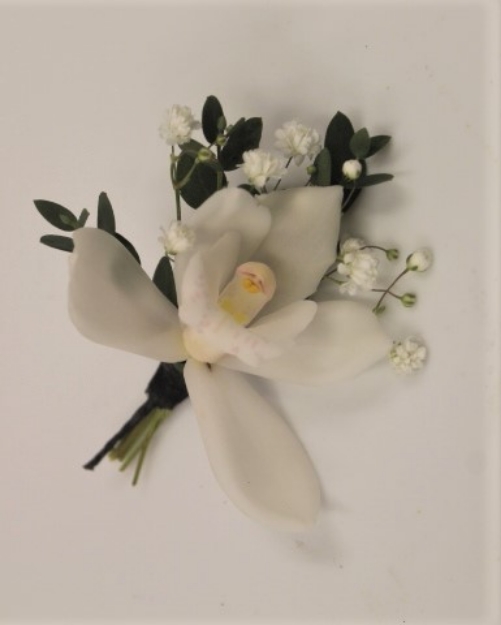The image captures a corsage-like arrangement centered within a vertical rectangular frame with a blended light gray and white background, reminiscent of a slight marble texture. Dominating the composition is a large white flower with oblong petals radiating from a cylindrical center that boasts hints of yellow and, subtly, purple. This prominent flower is angled towards the upper right, while its dark green stem and some lighter green stems point downwards to the lower left. Surrounding the main flower are clusters of smaller white flowers and buds, some still unbloomed, accompanied by dark and light green leaves that add to the floral ensemble. Shadows cast by the greenery enhance the depth against the white surface.